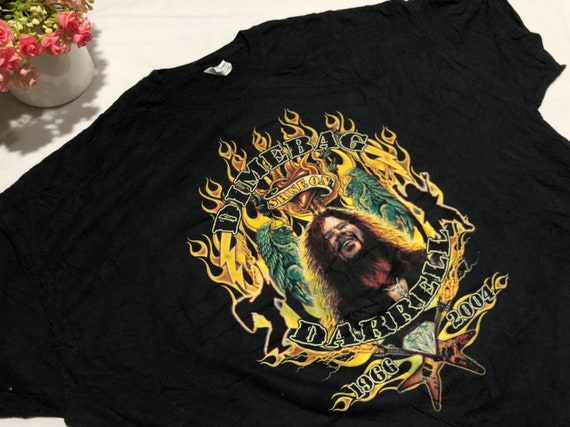This photo features a black t-shirt laid out on a white table, with a small potted plant in the background, containing green and pink flowers. The t-shirt prominently displays a detailed tribute to Dimebag Darrell. At the center, there is a vivid flame design encircling a portrait of Dimebag Darrell, captured with his long hair, mustache, and beard. The names “Dimebag” and “Darrell” are written in a circular fashion around the flames. The years 1966 and 2004 are displayed on either side of a diamond at the bottom of the graphic, signifying the years of his birth and death. Above the portrait, there’s a heart with a banner reading “Shine On.” The design also includes colors such as yellow, red, orange, and green, and features additional elements including silhouettes of dancing women within the flames, two guitars in an X pattern underneath the diamond, and what appear to be gargoyles and birds in the design.